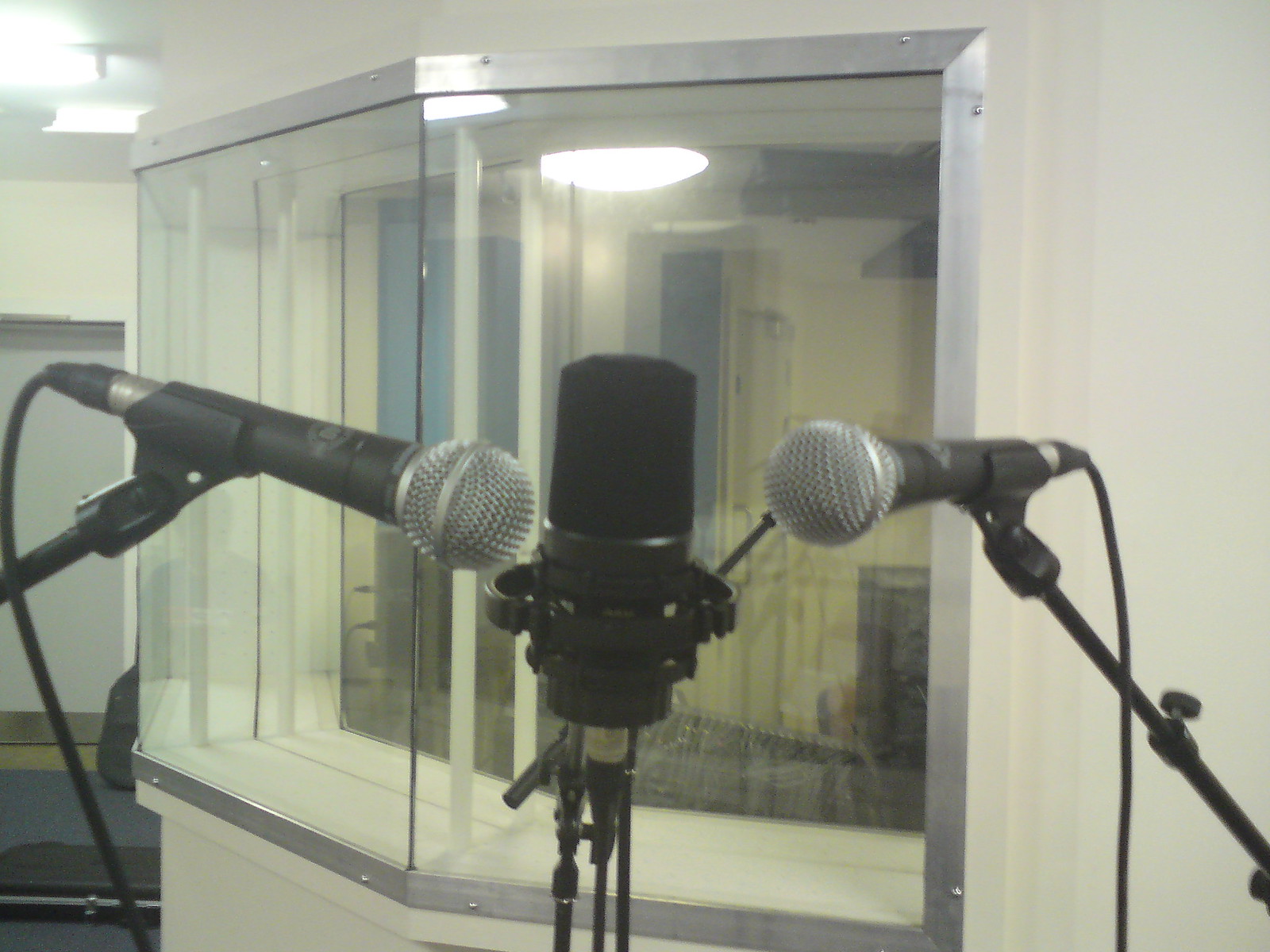The image is a brightly lit, indoor color photograph depicting a recording studio setup. In the foreground, there are three distinct microphones arranged together. The two outer microphones feature an elongated silver design, narrowing at their black clipped bases and expanding into a grey, meshed comb-effect head. These microphones are pointing towards the center. The central microphone contrasts with an upright, cylindrical black design, enclosed in a soft, fuzzy black cover and suspended in a black metal ring. All microphones are connected by wires to their respective stands.

Behind the microphones, the studio background includes white walls, possibly fitted with sound-dampening materials, and a multi-pane glass window with a silver trim on the left-hand side. This window separates the recording area from the control room, where sound engineers monitor and mix recordings. The room is illuminated with fluorescent white ceiling lights, casting a bright ambiance. Below, the floor is covered in dark blue carpet, and a case, likely for storing instruments, is partially visible in the bottom left of the image.